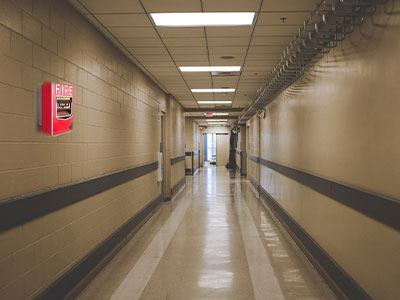The image captures a long, institutional hallway, possibly in a hospital, school, or mental institution. The corridor has a somewhat gloomy ambiance, with white-tiled ceilings featuring metal bars and water spouts for fire safety. Fluorescent lights illuminate the space from large openings in the ceiling. The walls on the left side are white cinder block, painted off-white with drab olive or dark green highlights at waist and ankle levels, while the opposite side is a lighter off-white drywall. Prominent on the left wall is a bright red fire alarm with a black handle and the word "FIRE" clearly visible. The floor tiles have a dark tan center bordered by a white line and edged with a darker tan. There is a pipe running down along the right side. Noteworthy details include a border-like railing running down the middle of the hallway and an exit sign above a door at the very end, where outside light filters through. The hallway seems to jog leftward towards its focal point, adding to its endless, mile-long appearance.